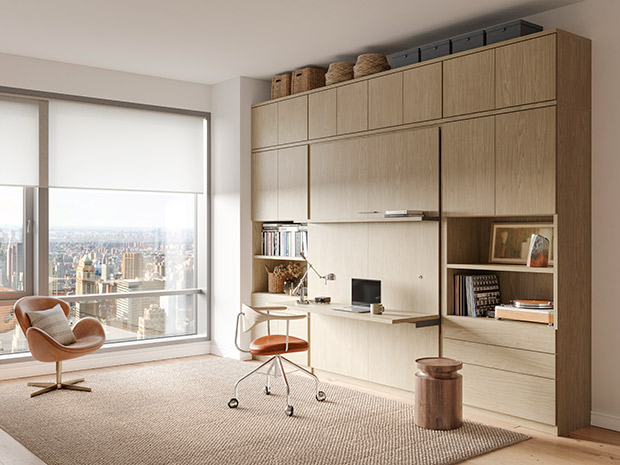The image is a full-color, square photograph taken indoors using natural light, capturing the detailed interior of a home office. The room is predominantly decorated in shades of white and light cream, complemented by a light brown wooden floor covered partially by a brown rug. A large window with a silver frame on the left side is mostly open, with shades pulled down about 20%, revealing a striking city skyline filled with tall skyscrapers.

The space features two distinctive chairs. To the bottom left, there is a stationary orange leather swivel chair with a white pillow, positioned near the expansive window. On the right side is a wooden desk area with numerous drawers and cabinets, some of which are closed, providing ample storage. The desk features a pulled-out shelf that serves as a standing desk, holding a laptop, a lamp, and a coffee mug. An office chair with wheels, characterized by an orange seat and a cream-colored backrest, is positioned at the desk.

Above the desk area is a large wall-mounted unit in light cream wood, functioning as a storage and display space. This unit includes two open shelves with books and decorative items, such as wicker baskets and possibly a metal jug. The shelving unit adds to the overall organized and inviting ambiance of this home office setting.